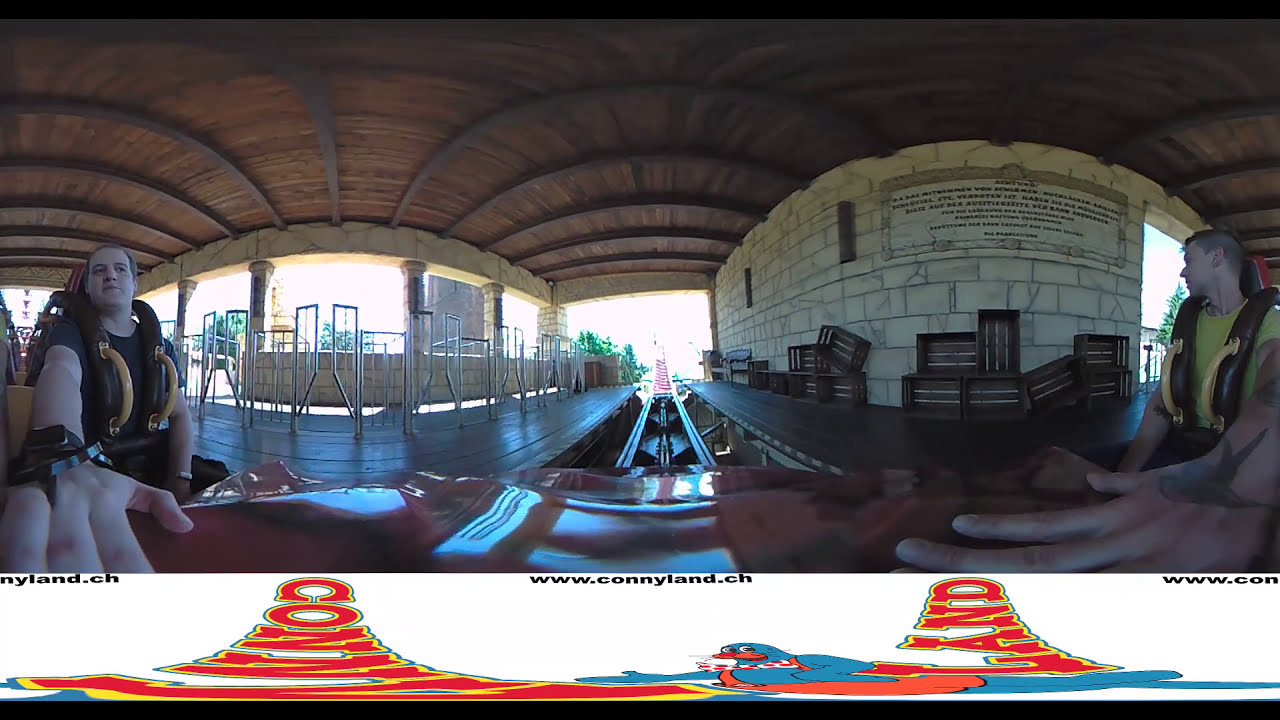This is a wide-angle color photograph of the interior of an amusement ride structure, likely at Connyland, a theme park indicated by the text "www.connyland.ch" found at the bottom center of the image. The scene is set inside a covered building with a rustic brown wood arched ceiling and features a pair of curved white brick walls toward the center right. The tracks, likely for a roller coaster or similar ride, run through the middle, flanked by sections of clear, window-pane structures.

In the photograph, two seated individuals are strapped into harnesses, suggesting they are on the ride. On the far left is an ambiguous Caucasian figure with light brown hair, wearing a brown vest with yellow metal handles. This person's right arm extends forward, but the hand is empty. On the right, a young Caucasian male with a closely cropped haircut, clad in a yellow t-shirt and a similar brown vest, is seen in profile. A left hand, possibly his, reaches into the foreground at the lower right corner. The image has a postcard-like, commercial quality, with additional text and a logo partially visible at the bottom, enhancing its advertisement nature.